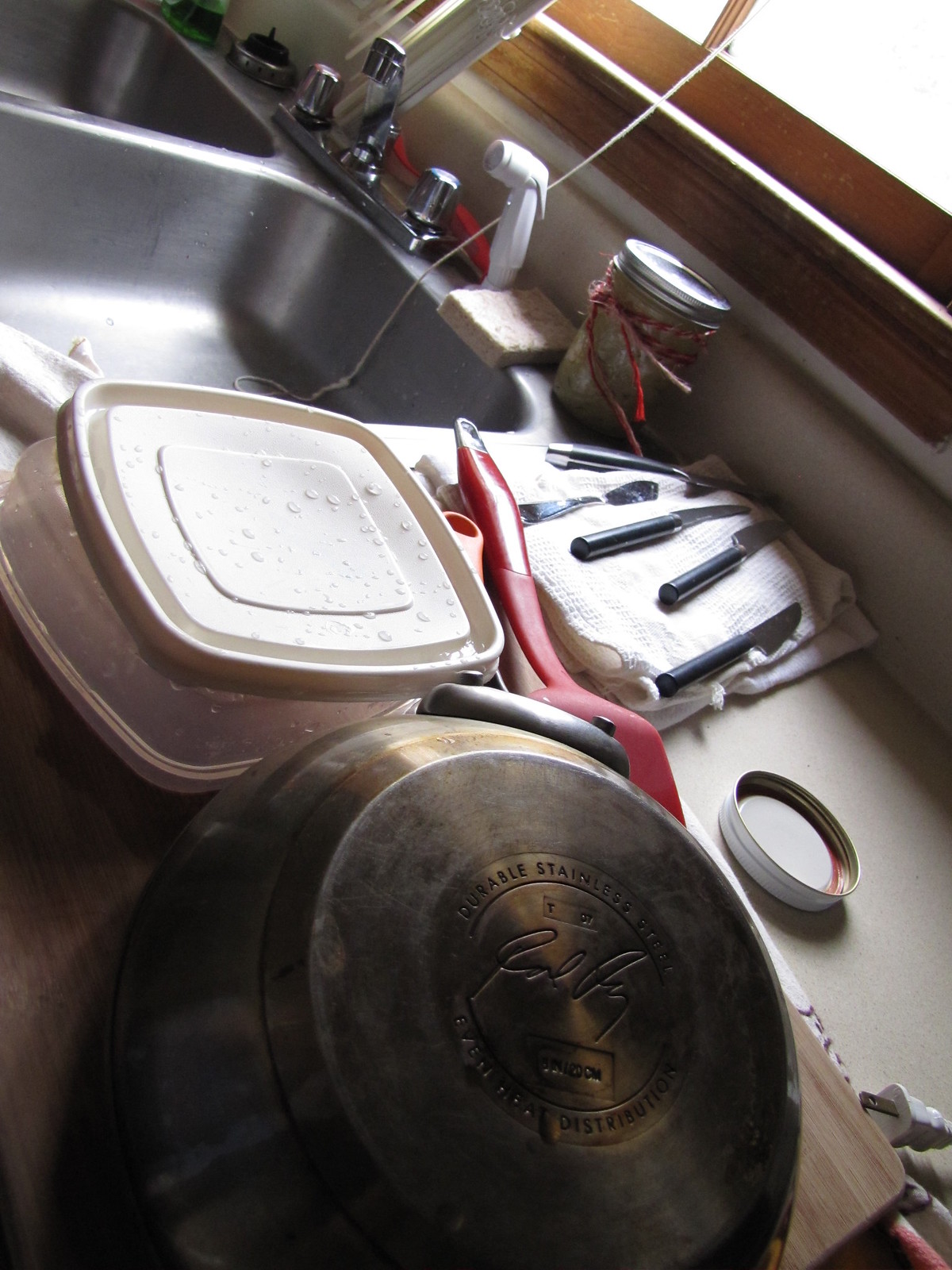This close-up, slightly tilted photograph captures a cluttered kitchen sink area. At the forefront, an upside-down durable stainless steel pot, featuring an indistinguishable autograph within a circular logo, dominates the scene. Adjacent to the pot, on the right, is the edge of a white cutting board and a jar lid. The white countertop beneath holds a white-bottomed Tupperware container with a clear lid, along with another white lid stacked on top. A red-handled spatula, also upside down, rests nearby. Toward the back, a hand towel spread out near the center-right supports a collection of drying knives. Beside the towel is a jar wrapped with a red string. The background reveals a silver sink equipped with matching faucet and knobs, accompanied by a white spray jet.